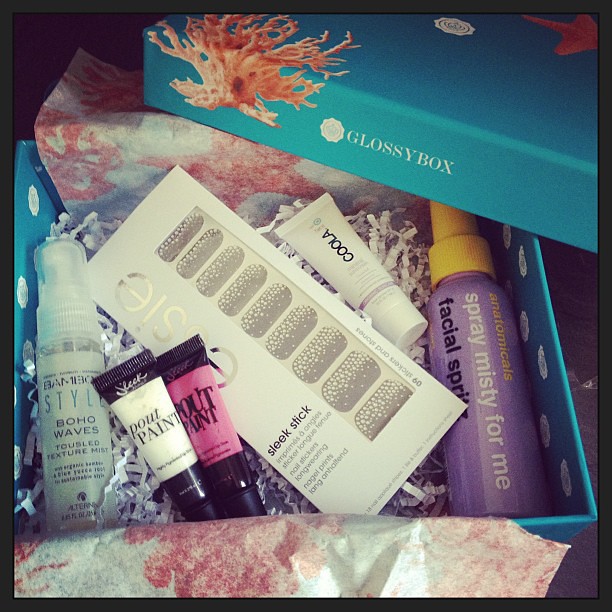The square image captures the meticulous arrangement inside a deep turquoise gift box with its lid slightly overlapping in the top right corner. The lid features a white logo and the text "Glossy Box" in white, along with a pink starfish in the top right and an orange coral illustration in the upper left corner. Inside the box, which is adorned with white polka dots and filled with protective white confetti, lies a collection of beauty products. On the left side rests a light green plastic container labeled "Style Boho Waves" with a white cap. To its right, there is a light purple bottle with a bright yellow cap that reads "Spray Misty for Me" in white text. Adjacent to this bottle, a smaller tube labeled "Coola" sits next to two compact tubes titled "Pout Paint" – one red with a black cap and the other white with a black cap, underneath which is a sleek, rectangular package of fake nails branded as "Sleek Stick". The careful presentation inside the box exudes a sense of luxury and thoughtful composition, making it a coveted gift for beauty enthusiasts.